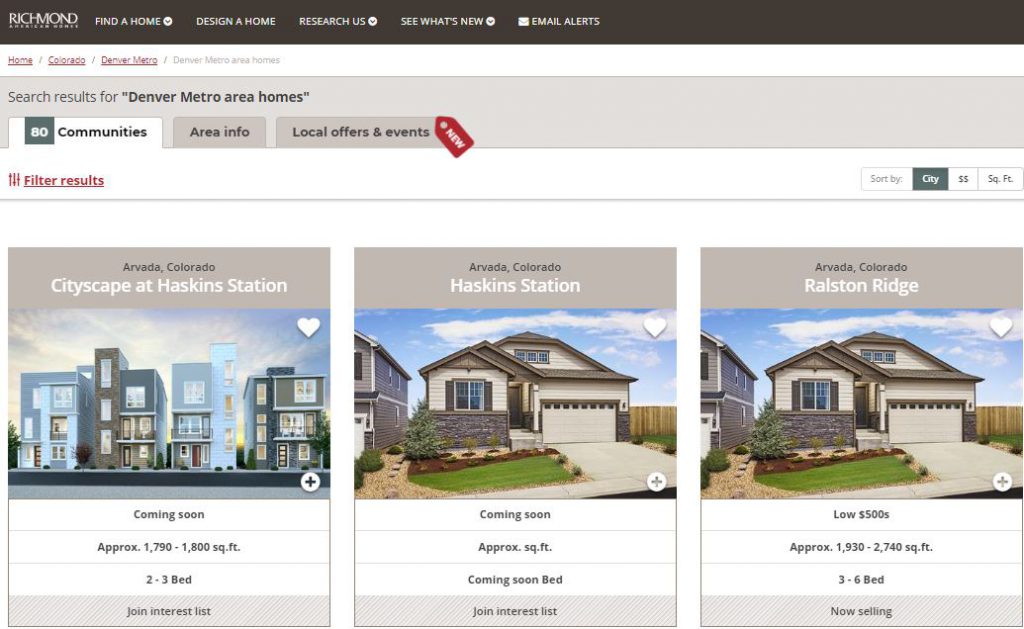The image features a dark brown banner running across the top with the word "Richmond" written in the left corner. To the right of this, there are buttons in white text labeled "Find a Home," "Design a Home," "Research Us," "See What's New," and "Email Alerts." Below this banner is a set of red links reading "Home," "Colorado," and "Denver Metro." 

Beneath these red links, there's a tan section with text that states "Search Results for Denver Metro Area Homes" and includes tabs labeled "80 Communities" (selected), "Area Info," "Local Offers," and "Events." Both "Local Offers" and "Events" tabs have a red tag that says "New." 

Further below, the background transitions to white, displaying four images of homes. The first image on the left shows townhomes and includes the text: "Arvada, Colorado - Cityscape at Haskin Station - Coming Soon - Approximately 1,790 to 1,800 square feet - 2 to 3 Bedrooms - Join Interest List." 

The middle image depicts a two-story single-family detached home labeled: "Arvada, Colorado - Haskin Station - Coming Soon - Approximate Square Foot (blank) - Coming Soon - Bed - Join Interest List."

The rightmost image is a repeat of the middle home, but labeled with: "Arvada, Colorado - Ralston Ridge - Low 500s - Approximately 1,930 to 2,740 square feet - 3 to 6 Bedrooms - Now Selling."

The overall layout provides a clear and organized presentation of the homes available in the Denver Metro area, with detailed information about each property and options to join interest lists or view more details.